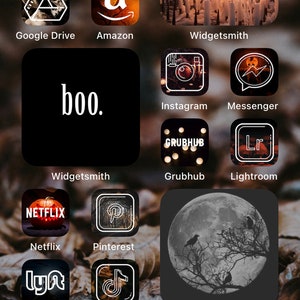This detailed caption provides a thorough description of the screenshot from an iPhone’s homepage. It aims to offer a clear image of the arrangement and appearance of the apps and widgets:

---

The image is a small screenshot of an iPhone’s homepage running on the iOS platform. The apps and widgets are organized in a grid pattern, against a predominantly dark-colored background featuring an outdoor scene, likely depicting leaves or trees, though it is slightly out of focus.

A total of ten popular apps are visible, each with a square icon. In the top left corner, we have Google Drive and Amazon. Centrally to the right, there are Instagram, Messenger, Grubhub, and Lightroom apps. The bottom left corner showcases Netflix, Pinterest, Lyft, and TikTok.

Three larger widgets, each occupying the space of four app icons, are also present. In the top right corner is a Widget Smith widget with an orange or brown background, partially out of view. Another Widget Smith widget is located in the center left, featuring a black box with white text that says “Boo.” The bottom right widget displays an image of a light gray moon with trees and birds overlaid on a dark gray background, though its name is not visible.